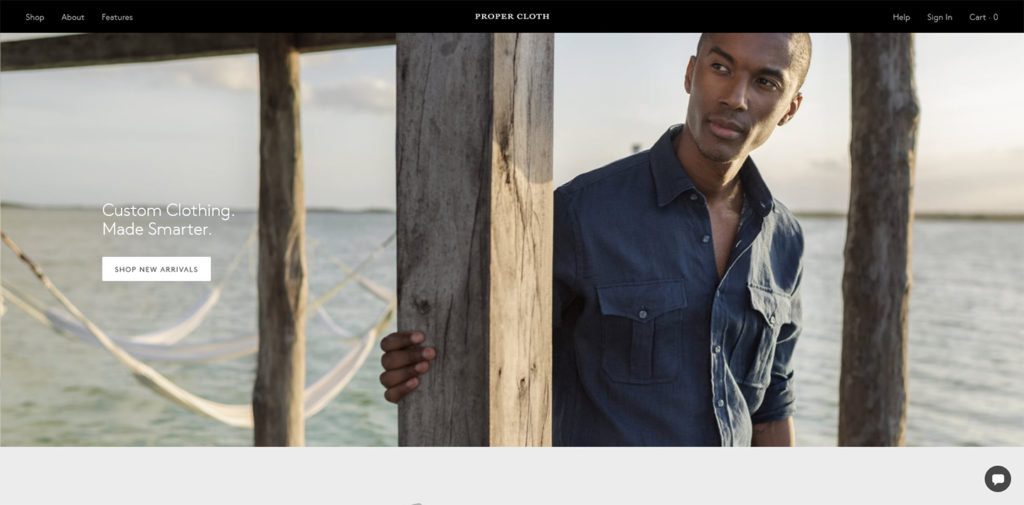The image features a webpage with a black header at the top. Centered in the header, white text reads "Proper Cloth." On the top left, there are navigation tabs labeled "Shop," "About," and "Feature." On the top right, options for "Help," "Sign In," and "Cart" (indicating zero items) are present. 

In the main section of the image, on the left side, white text declares, "Custom clothing made smarter." Below it, there are three buttons: "Shop," "New Arrivals," and a third white button with black text. 

On the bottom right corner of the image is a black chat icon labeled "Chat with us." 

At the center of the image stands a person wearing a dark blue t-shirt, leaning against a brown wooden pillar with dark textures. This pillar is one of three, supporting a horizontal wooden beam extending to the left. 

In the background, a lake with dark green water is visible, bordered by a stretch of green land. The background is slightly blurry, adding depth to the scene. To the left side of the image, there is a small white object. The person in the dark blue t-shirt is facing towards the left side of the image.